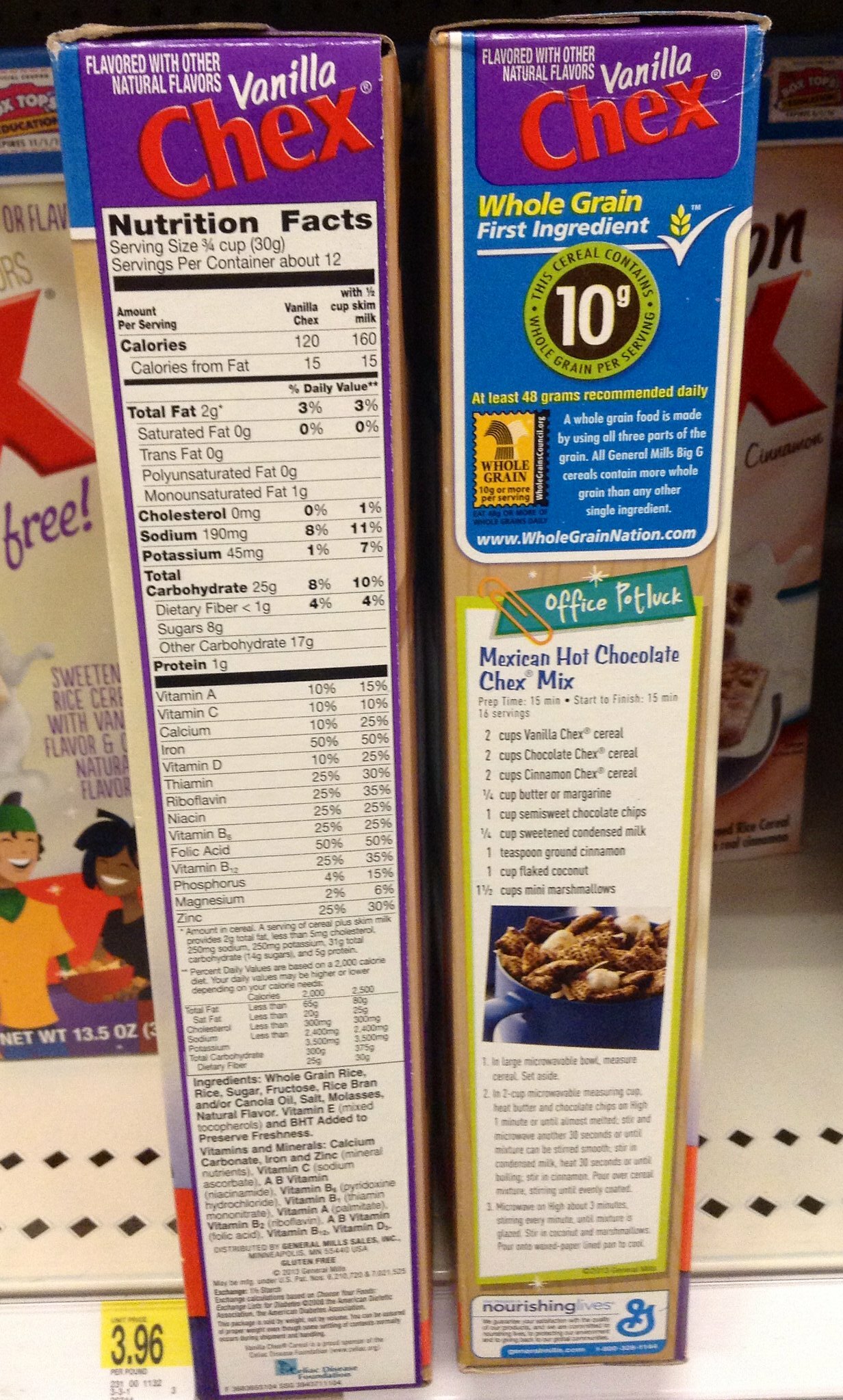This vertically cropped color photograph captures an organized supermarket shelf, holding two boxes of Vanilla Chex cereal prominently displayed. The shelf itself is constructed of off-white metal, typical of retail shelving. The two focal boxes are positioned edge-on, with the left box showcasing nutritional information, including vitamins and ingredients, on its vertical side. Adjacent and surrounding these boxes are additional identically branded Vanilla Chex boxes arranged in neat rows.

The right-side box stands out with its detailed front design. At the top center, a recognizable blue background hosts the Vanilla Chex logo. Just below, the majority of the box's front is dedicated to a detailed recipe for "Mexican Hot Chocolate Chex Mix," enticing shoppers with a flavorful suggestion. The bottom section of the box features the colorful General Mills symbol, adding brand credibility and visual appeal. The image is brightly lit by artificial store lighting, enhancing the vivid colors and fine details of the packaging, highlighting the appealing presentation typical of supermarket products.